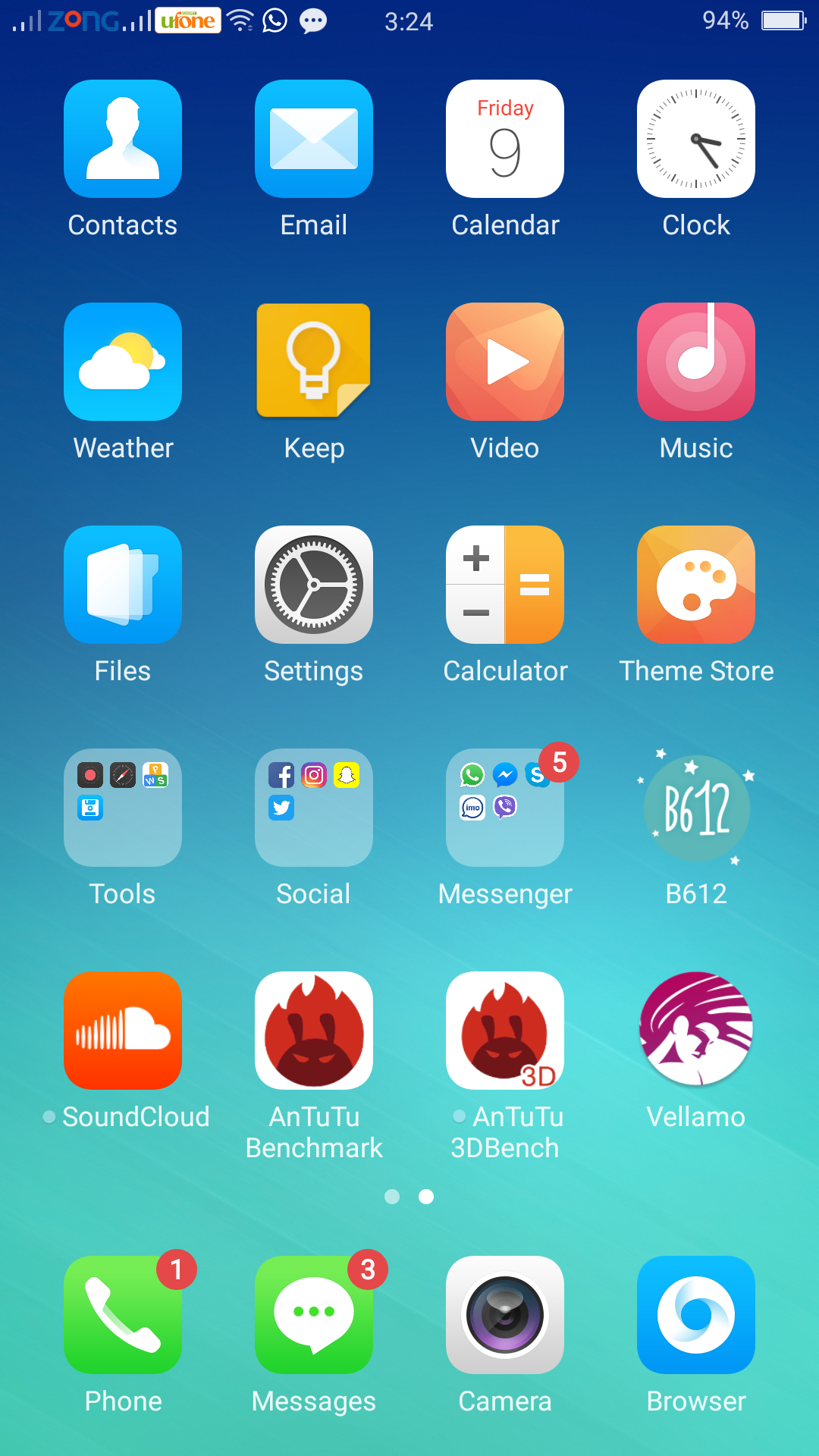Here is a cleaned-up and detailed caption for the image described:

---

This is a screenshot of a cell phone screen displaying its home interface. The background at the top is a dark blue that smoothly transitions into a lighter blue, and finally merges into a seafoam green at the bottom. In the upper right-hand corner, there's a battery icon with its percentage next to it. The upper left-hand corner shows signal strength and Wi-Fi indicators.

The screen is organized into a grid of icons, featuring four icons across and six rows down. Each icon represents a different app or function, housed within a square icon.

From top to bottom, left to right, the icons are arranged as follows:

1. **Contacts** - represented by a contact book icon.
2. **Email** - depicted with an envelope icon.
3. **Calendar** - symbolized by a calendar icon.
4. **Clock** - shown with a clock face icon.

In the second row:
1. **Weather** - indicated by a weather-related icon.
2. **Keep** - represented by a lightbulb icon often associated with Google Keep.
3. **Video** - symbolized by a play button icon.
4. **Music** - depicted with a musical note icon.

The third row features:
1. **Files** - indicated by a folder icon.
2. **Settings** - depicted with a gear icon.
3. **Calculator** - symbolized by a calculator icon.
4. **Theme Store** - represented by a paintbrush or palette icon.

On the fourth row:
1. **Tools** - possibly represented by a toolbox icon.
2. **Social** - depicted by an icon representing social media or communication apps.
3. **Messenger** - symbolized by a chat bubble icon.
4. **B612** - denoted with its specific branding icon.

In the fifth row:
1. **SoundCloud** - represented by the SoundCloud logo.
2. **AnTuTu Benchmark** - denoted by its specific branding icon, with uppercase letters "A" and "T" followed by "U" in a pattern.
3. **AnTuTu 3D Bench** - similarly represented by its branding icon.
4. **Vellamo** - symbolized by the Vellamo logo.

Finally, in the last row:
1. **Phone** - indicated by a traditional phone receiver icon.
2. **Messages** - depicted with a chat bubble icon.
3. **Camera** - symbolized by a camera lens icon.
4. **Browser** - shown with a globe icon, representing internet browsing.

---

This detailed caption provides a comprehensive visual description of the cell phone screen screenshot.